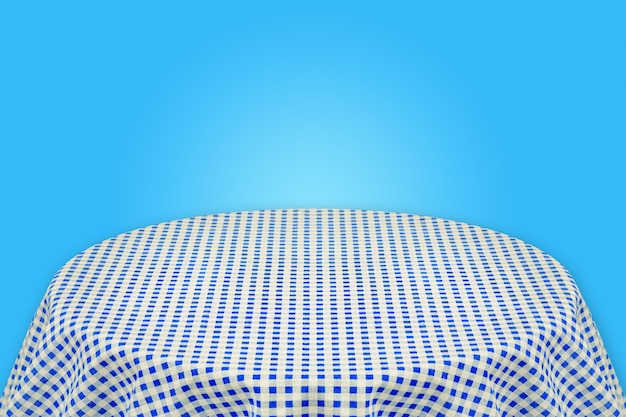The image depicts a simple yet detailed scene of a round table adorned with a checkered tablecloth. The tablecloth features a bright royal blue and white gingham pattern, which subtly wrinkles as it drapes over the table's circular edges. The background of the photograph is a smooth, sky blue with a turquoise tint, brighter in the center and fading towards the edges. This blue backdrop forms a striking contrast with the vibrant checkered design of the tablecloth, enhancing the overall visual appeal. The photograph is rectangular, slightly longer in width, capturing the serene simplicity and color harmony of the scene, with no other objects present to distract from the central focus on the tablecloth and the complementary hues of blue.